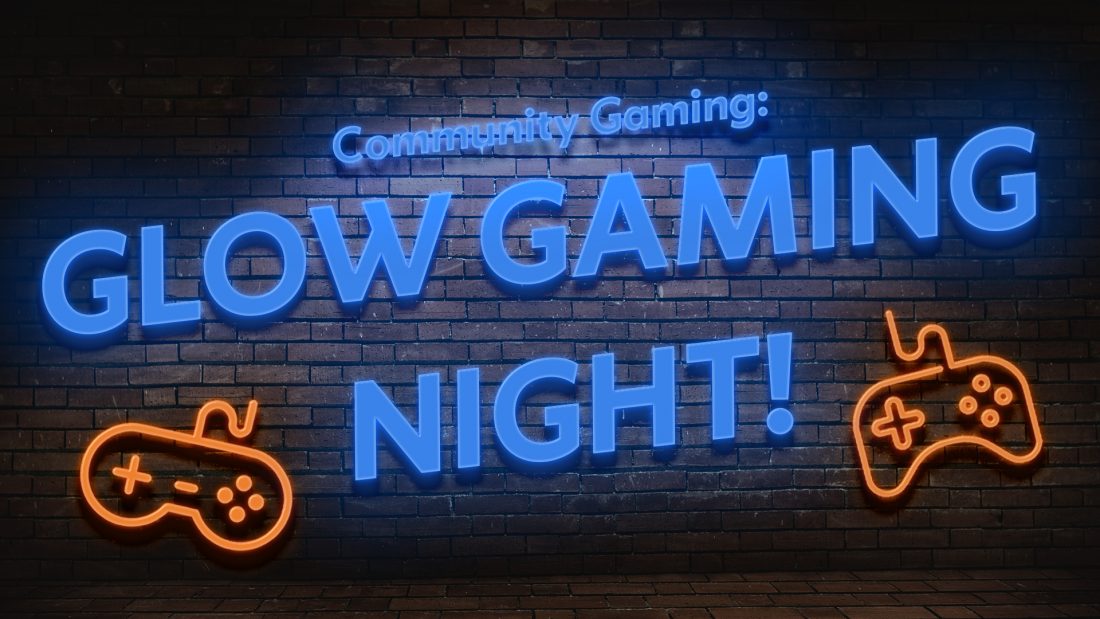This digital poster promotes a game night titled "Glow Gaming Night!" The background features a grayish-black brick wall, illuminated by a spotlight, adding a subtle glow. At the top, in smaller neon blue text, it reads "Community Gaming." Below that, in large block letters also in neon blue and angled slightly upward from left to right, the text proudly announces "Glow Gaming Night!" with an exclamation point. Flanking the word "night" are two neon orange outlined game controllers. On the left side is a retro Super Nintendo controller with its characteristic rounded edges and four buttons, complete with a little cord. On the right side is a more modern PlayStation controller, identifiable by its ergonomic handles and button layout. The vibrant neon colors against the dark brick backdrop create a striking and inviting advertisement for the event.